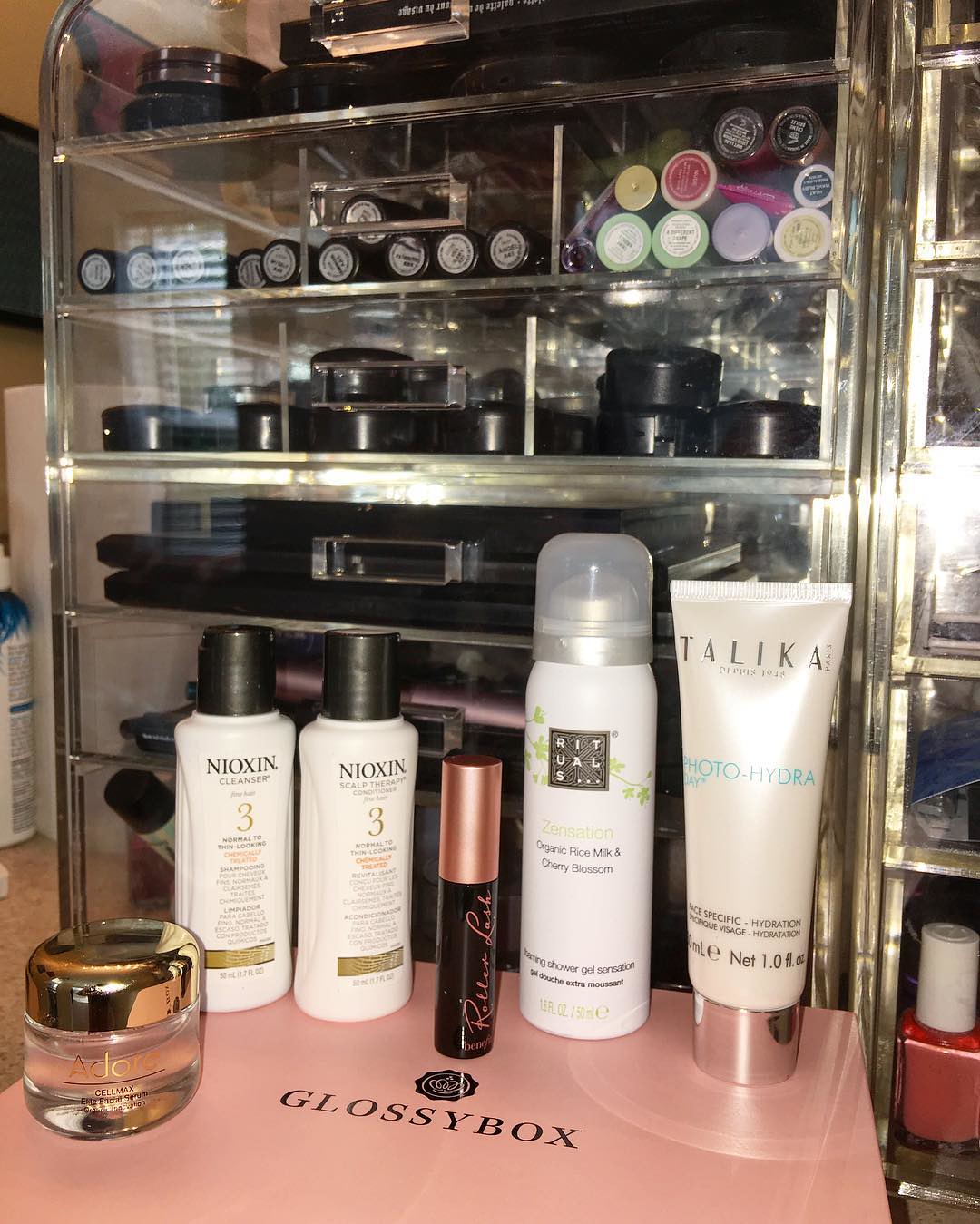The image captures a well-organized, clear acrylic makeup stand. The stand features six distinct rows of compartments, ascending vertically. The very top row is partially obscured but houses several black containers. The second row showcases an assortment of lipstick tubes, varying in both color and label. These include black tubes with white labels and other tubes in black, yellow, purple, red, and light green. The third and fourth rows are arranged with more uniform black containers, while the fifth row includes black containers accompanied by some pink items. The contents of the sixth row remain out of view due to a series of bottles placed in front of it.

In front of the stand, on a pink box labeled "Glossy Box," a clear container with a gold top is prominently displayed. Accompanying it are two white bottles labeled "Nioxin 3," distinguished by their black tops. Additional items include a black tube with a rose gold cap, a white mousse bottle with a clear rounded cap, and a cream tube capped with silver. The meticulous arrangement and variety of cosmetics make for an aesthetically appealing and organized display.